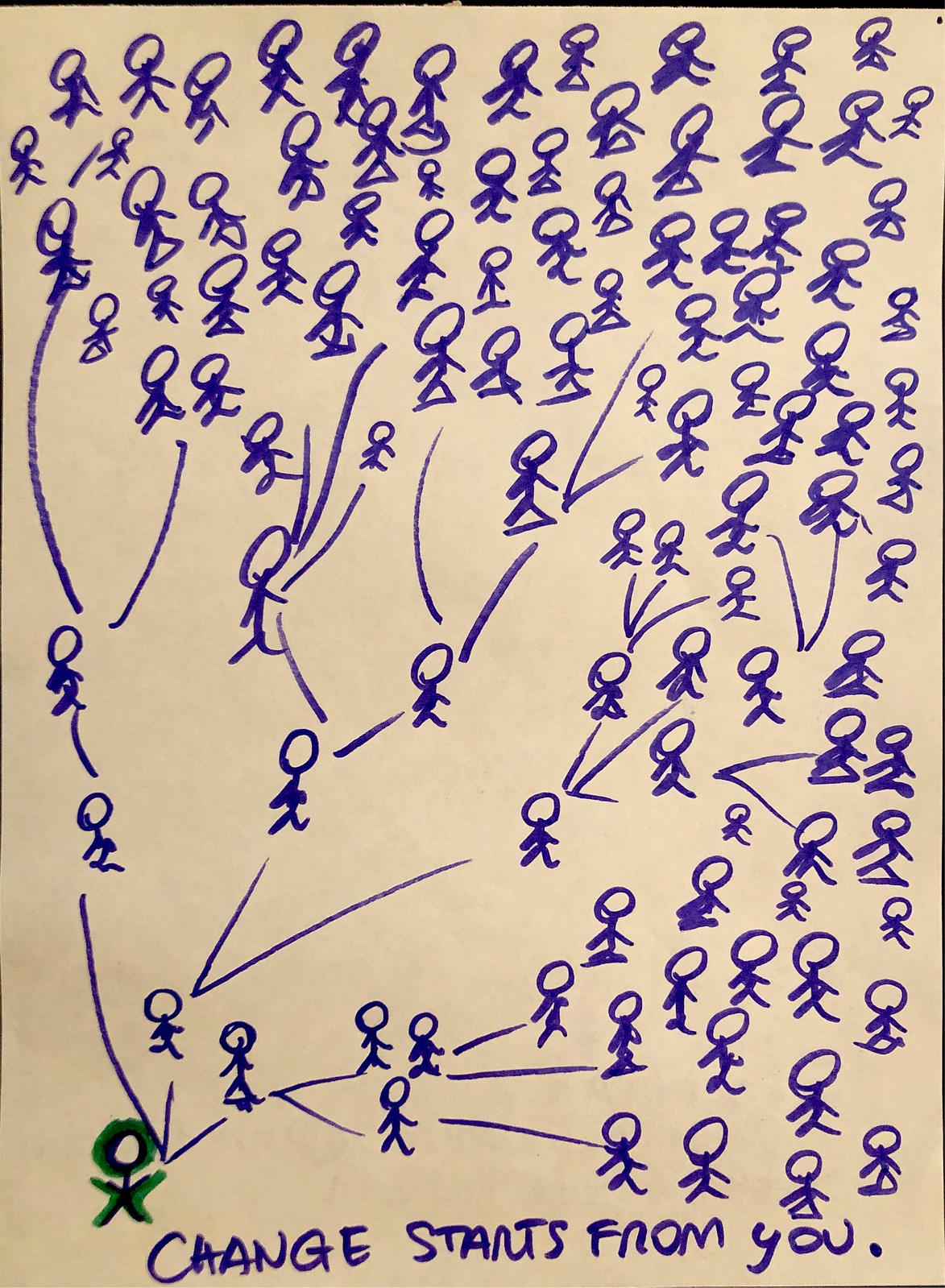The image depicts a densely packed array of blue stick figure people drawn on a white piece of paper. At the bottom of the page, prominently displayed in bold blue capital letters, is the phrase "CHANGE STARTS FROM U." In the lower left corner, a single stick figure, distinguished by being drawn in green marker, stands out. Radiating from this green stick figure are several arrows extending in different directions. These arrows lead to smaller blue stick figures, suggesting a chain reaction. The visual narrative implies that the actions of the individual in green influence multiple blue stick figures, who in turn influence even more individuals, creating a cascading effect that spreads across the entire page. The style of the drawing, along with the distribution of the figures, emphasizes the concept of individual impact on broader change. The paper itself rests on a brown surface, indicated by the thin brown border visible around its edges. The absence of other text ensures that the viewer's focus remains on the interconnected web of figures and the central message.